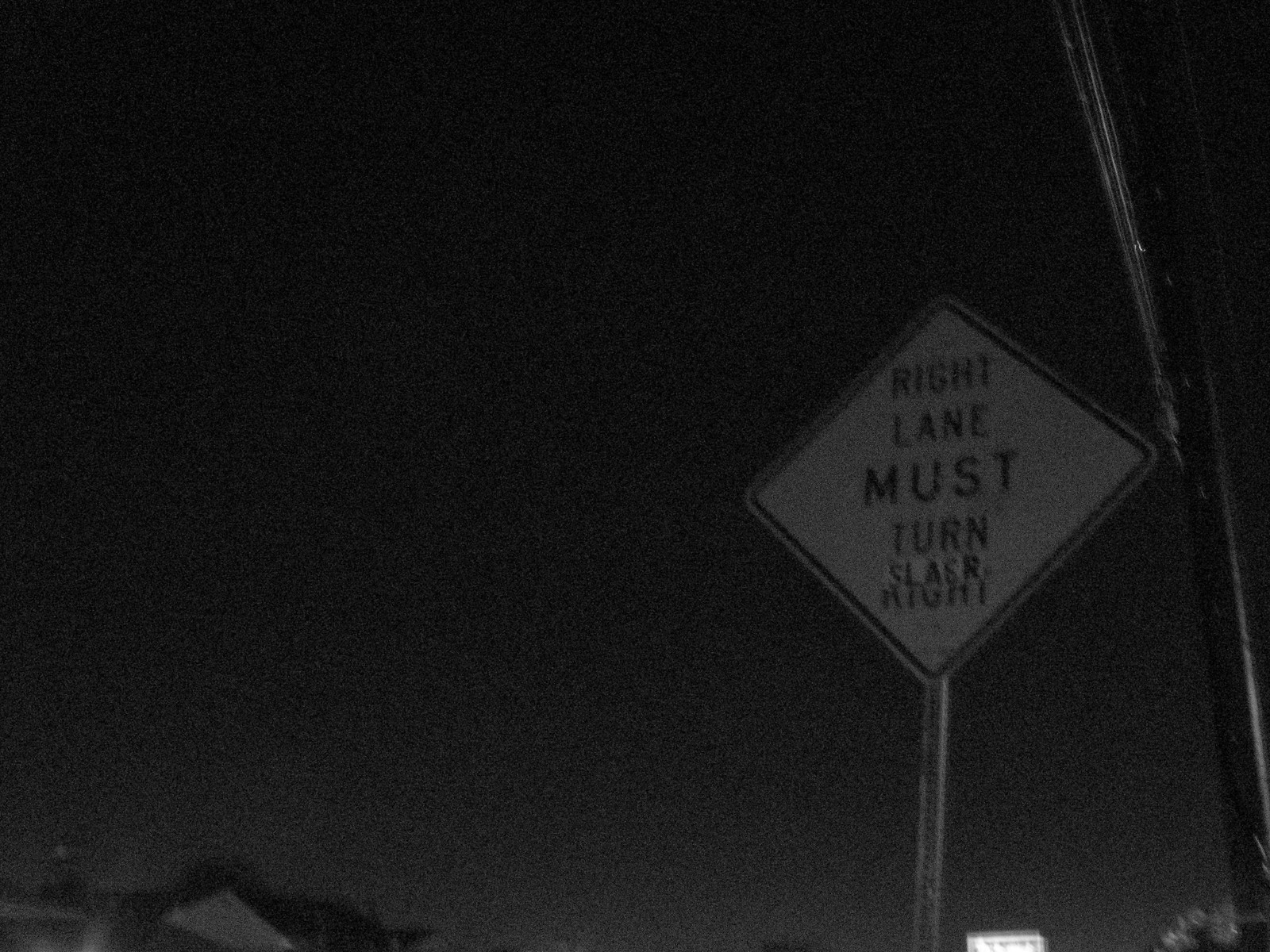The image, wider than it is tall, captures a dimly lit nighttime scene. A subtle gradient at the bottom lightens the darkness slightly. On the right-hand side, a street sign ascends from the lower edge of the frame, declaring "Right Lane Must Turn." However, the word "Right" has been defaced and replaced with "S-L-A-S-R," suggesting someone has tampered with the sign. The lower left-hand corner holds some indiscernible small objects. Along the right edge of the image, a linear element that might be a windshield wiper or another obscure object is visible, hinting that the photo could have been taken through a car window. Completing the scene, a small, bright box appears in the bottom right corner, its purpose or identity unclear.